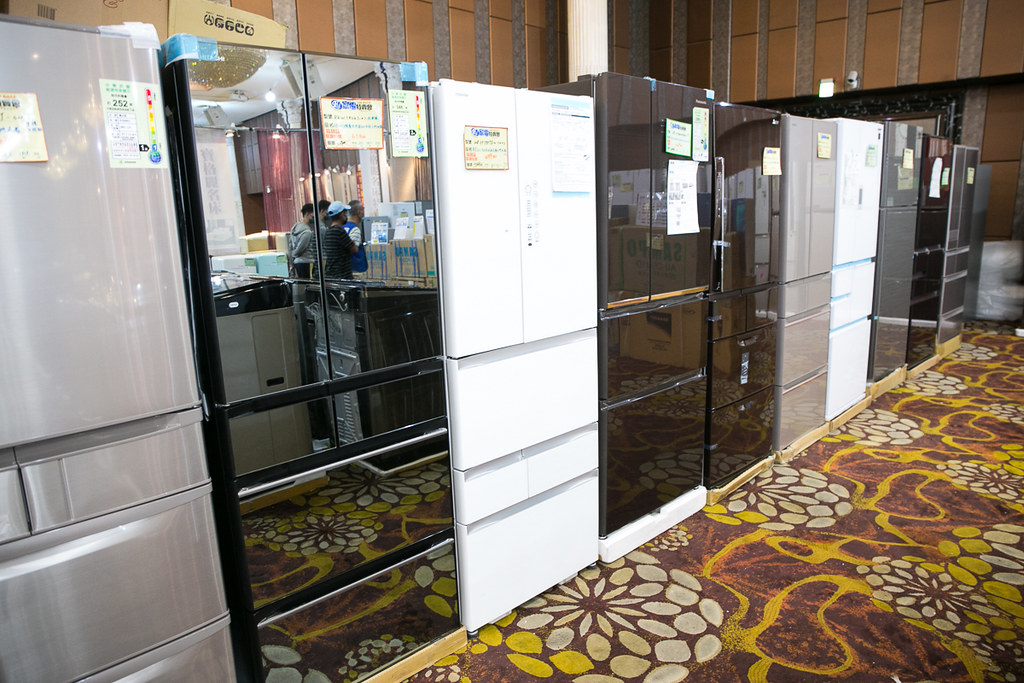The image captures the interior of an appliance store showcasing a neat row of various refrigerators. The eye is immediately drawn to the garish flooring, which features a rust brown carpet with yellow swirling lines and white flower petal patterns prevalent across it. The refrigerators, all neatly aligned from the left to the right side of the photo, display a variety of finishes—ranging from glossy black and silver to white. Each refrigerator is still partially wrapped in protective film and stands on what remains of their packaging bases, which often consist of rigid cardboard or styrofoam. Notably, these refrigerators exhibit modern designs with multiple compartments, including two bottom drawers and French doors at the top.

The left side of the image suggests division into smaller sections using alternating panels of smoky colored glass and solid gray-white rectangles that extend upwards but do not reach the ceiling. This partitioning gives the space a modular look, akin to small private rooms akin to safety deposit box rooms in a bank.

In the upper part of the image, the brown-striped wallpaper with textured, silver panels defines the upper sections of the walls. The wallpaper transitions into a tan checkered design with wooden panel inserts, creating a vintage ambiance in the store. The combination of retro flooring and modern appliances presents a striking visual contrast.